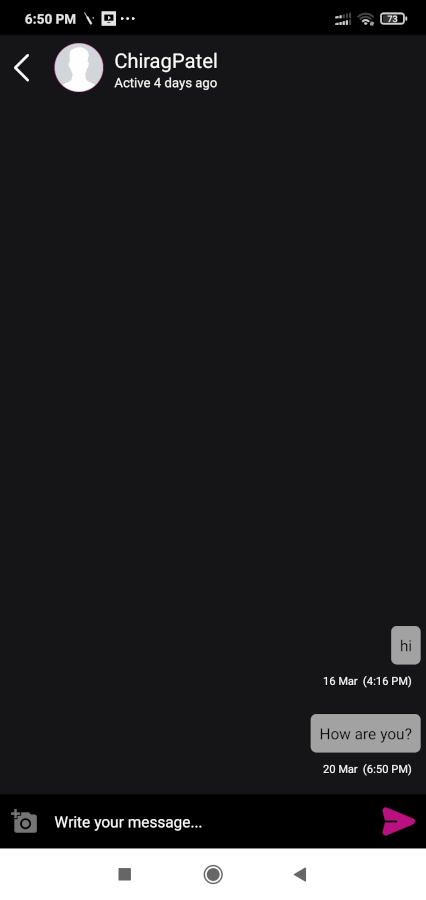This image is a screenshot of a cell phone displaying a messaging app interface. The main background of the app is a dark gray, with a thinner black strip at the very top where cell phone status icons are located. On the upper left-hand corner of the screen, there is a white back arrow. The top of the message area features contact information showing the name "Chirag Patel" and an "active 4 days ago" status.

The conversation contains two messages:
1. The first message reads, "Hi."
2. The second message reads, "Hi. How are you?"

At the bottom of the screen, there is a text input box where users can type their messages. This input area is black, and there is a gray picture icon on the lower left side of this box. On the lower right side, there is a pink send button depicted as a right-pointing arrow.